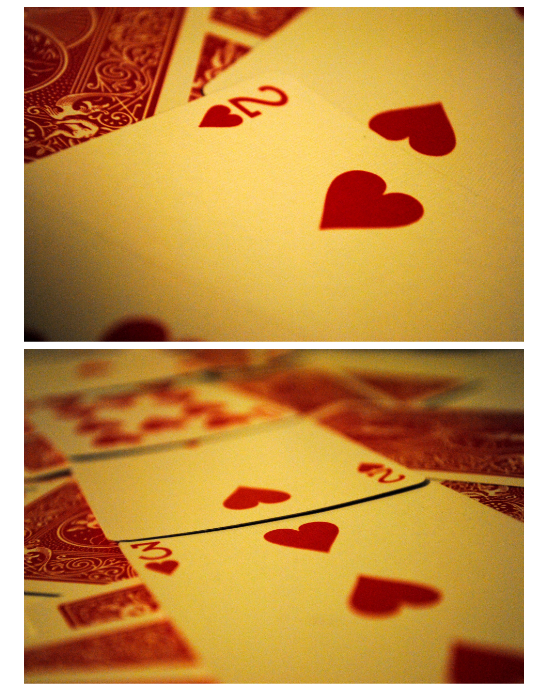This image features two photographs of playing cards, stacked one above the other. The top photograph showcases a two of hearts prominently, partially obstructing another heart card whose number remains obscured. In the background of this photo, additional playing cards are visible, displaying red backs adorned with intricate designs. The face side of the visible two of hearts card is a light beige color, marked with the numeral "2" and a large heart symbol.

The bottom photograph displays a diagonally arranged, face-up row of playing cards starting from the lower right and extending to the upper left. This row includes a three of hearts, a two of hearts, and another heart card with an indistinct number. Beneath this line of face-up cards, several other cards lie face-down in a haphazard arrangement. The three of hearts card is detailed with a small numeral "3" adjacent to a heart symbol, and three larger hearts—a single heart oriented upside down, flanked by two upright hearts.